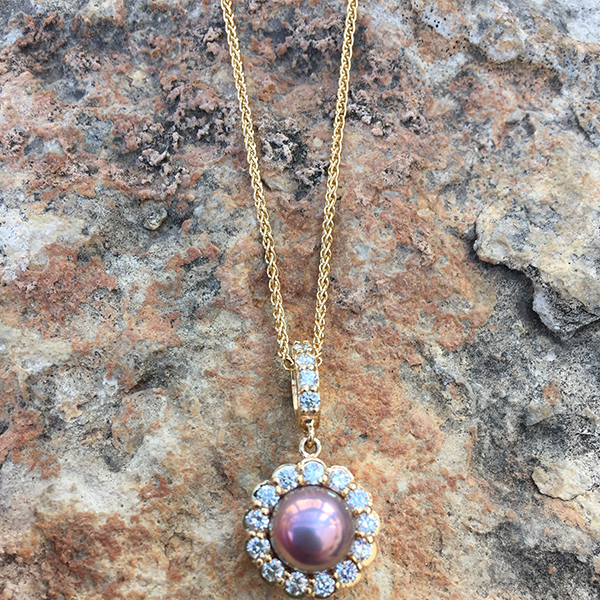The image captures a detailed photograph of an antique-style, delicate gold necklace displayed against a textured, rough, and ridged rock surface. The rock forms the entire background, presenting an interesting blend of orangish, dark gray, and light gray hues. The necklace's chain appears to loop like a bracelet, showcasing a classical elegance. The centerpiece of the necklace is the main focus—a large central pearl with a pinkish hue, enveloped by sparkling diamonds. Attached above the pearl, a small segment adorned with more diamonds connects to the chain. The pendant's base consists of two interconnected rings, each set with blue gemstones, encircling a central purplish-colored spherical gem, enhancing the intricate and luxurious design.